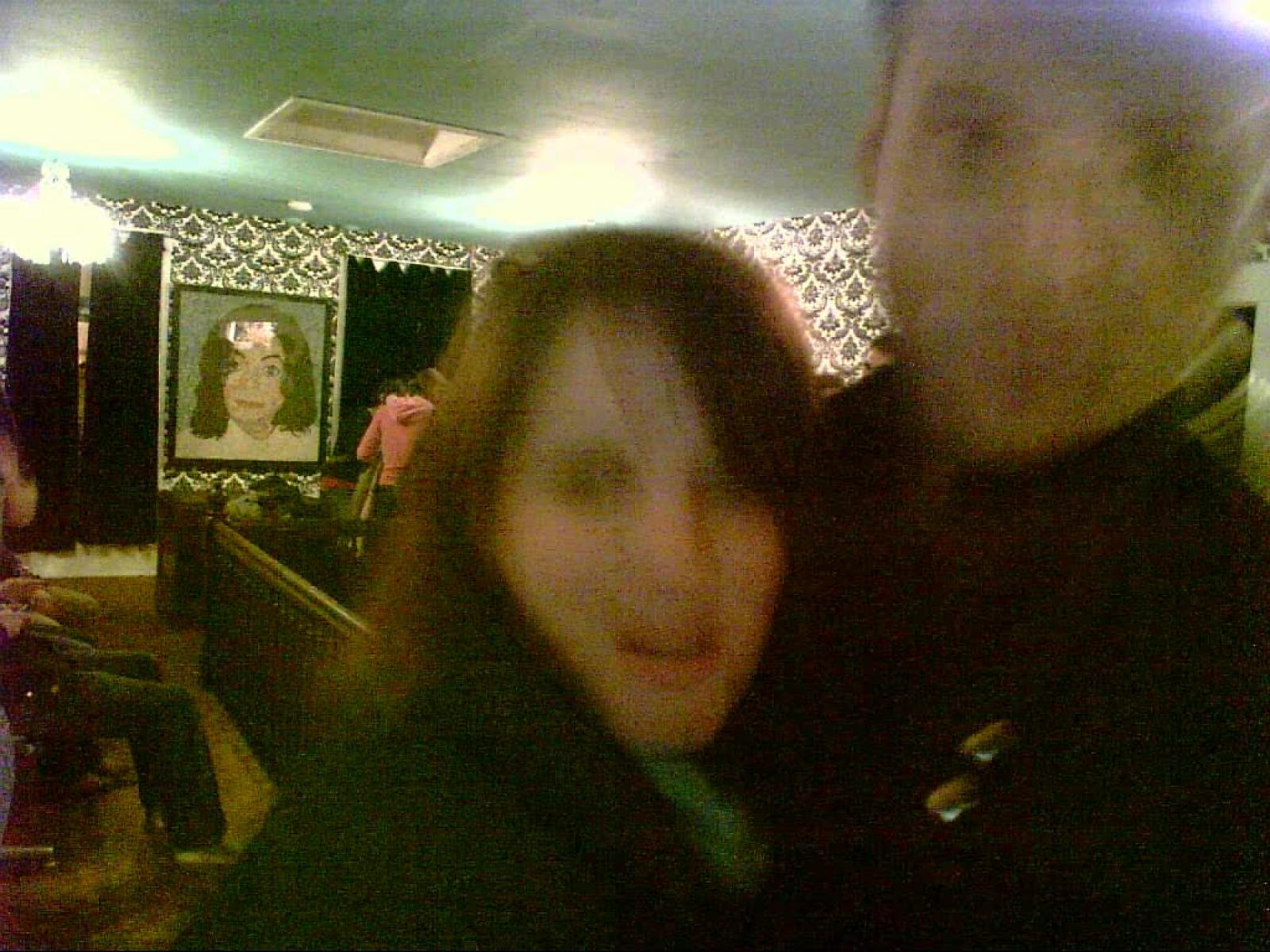This rectangular image depicts a very blurred, low-resolution indoor scene. On the right half of the image, a couple stands close together, captured from the chest up. The female has fair skin and long brown hair swept to the side, and she is dressed in a dark-colored shirt or jacket. Standing to her right is a taller male, also with fair skin and wearing a dark jacket. Due to the poor quality of the photo, their facial features and eye colors are indiscernible. 

In the background, the indoor setting reveals chairs along the left wall, occupied by unidentified individuals, with only their legs visible. The back wall is adorned with a busy black-and-white patterned wallpaper, where a framed artwork of Michael Jackson is prominently displayed. The artistic portrayal of the legendary pop singer adds a focal point to the chaotic backdrop.